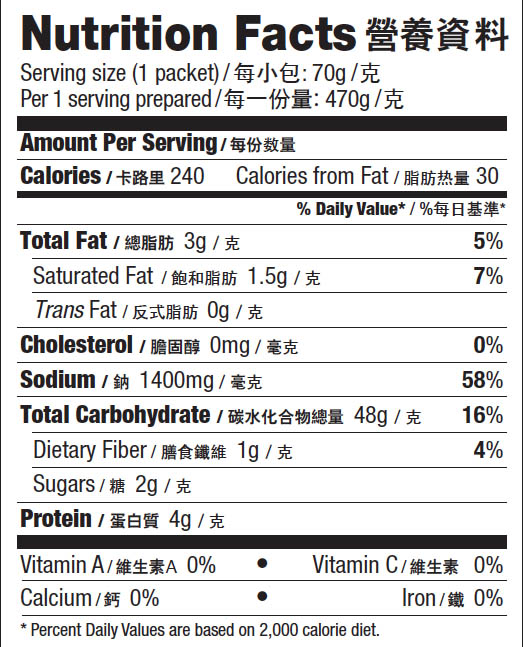The image depicts a meticulously scanned nutrition label, featuring both English and Chinese text, neatly formatted with black-bordered and columned rows on a white background. At the top, it prominently states "Nutrition Facts" followed by its Chinese translation. The serving size is listed as "one packet per serving" with a weight of 470 grams. Below this, detailed nutritional information includes: 240 calories per serving, with 30 calories from fat. The breakdown shows 3 grams of total fat (5% DV), including 1.5 grams of saturated fat (7% DV) and no trans fat. Cholesterol is listed at 0%, sodium at a significant 1400 milligrams (58% DV), total carbohydrates at 48 grams (16% DV), dietary fiber at 1 gram (4% DV), sugars at 2 grams, and protein at 4 grams. The vitamins and minerals section notes that there is 0% of Vitamin A, Vitamin C, calcium, and iron. An asterisk at the bottom indicates that the daily values are based on a 2,000 calorie diet.